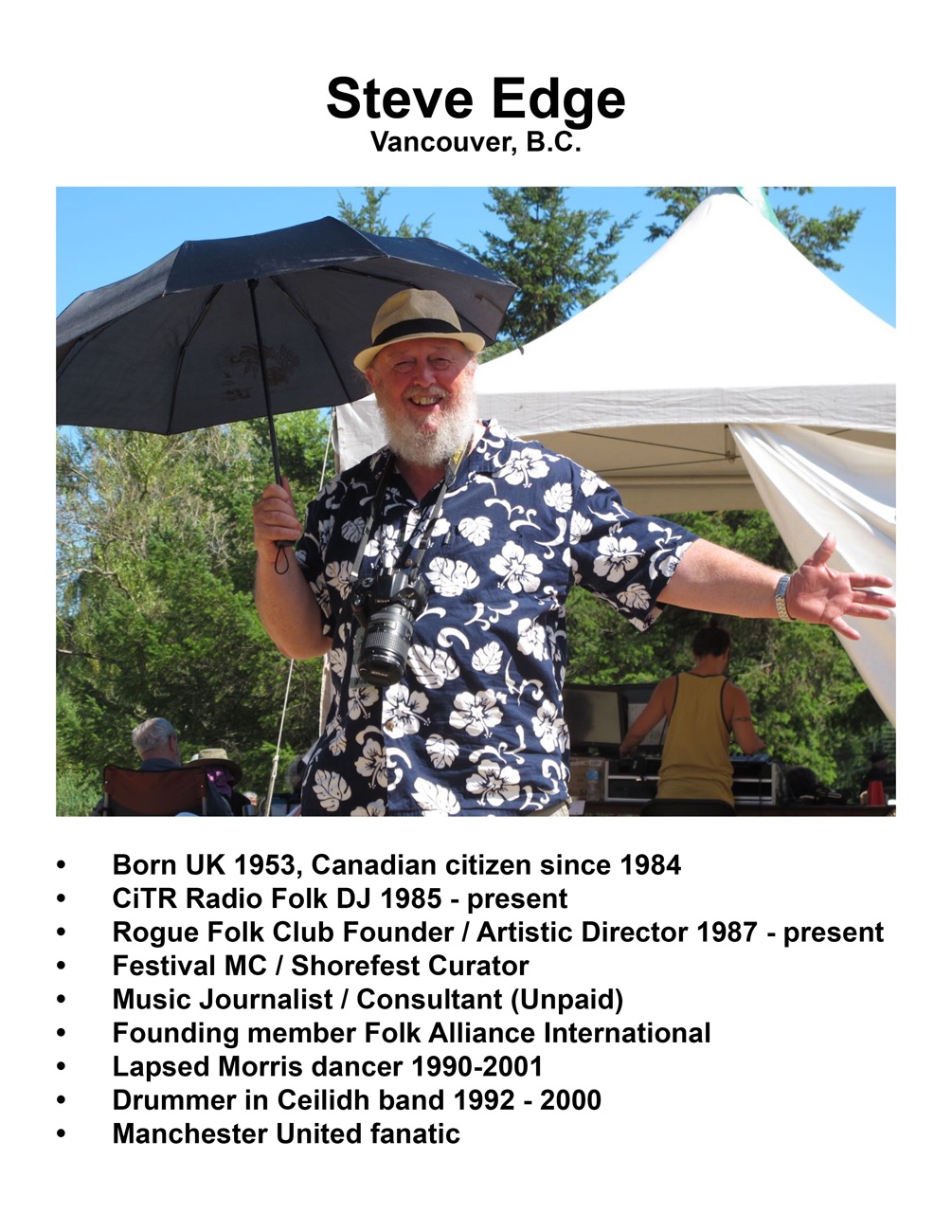In this detailed photograph, a smiling white man with a white beard, identified as Steve Edge from Vancouver, BC, stands under a bright sun, shielding himself with a black umbrella held in his right hand. He is sporting a tan-brimmed hat with a black band and a navy blue Hawaiian-style shirt adorned with white floral patterns. Around his neck hangs a camera, and he has a watch on his left wrist. He stands in front of a white event tent, with another person partially visible in the background. The image is complemented by black text on a white background, summarizing Steve's life and career: "Born UK, 1953, Canadian citizen since 1984, CITR Radio Folk DJ, 1985-present, Rogue Folk Club Founder Artistic Director, 1987-present, Festival MC, Shorefest Curator, Music Journalist Consultant (Unpaid), Founding Member of Folk Alliance International, Lapsed Morris Dancer, 1990-2001, Drummer in Ceilidh Band, 1992-2000, Manchester United Fanatic."